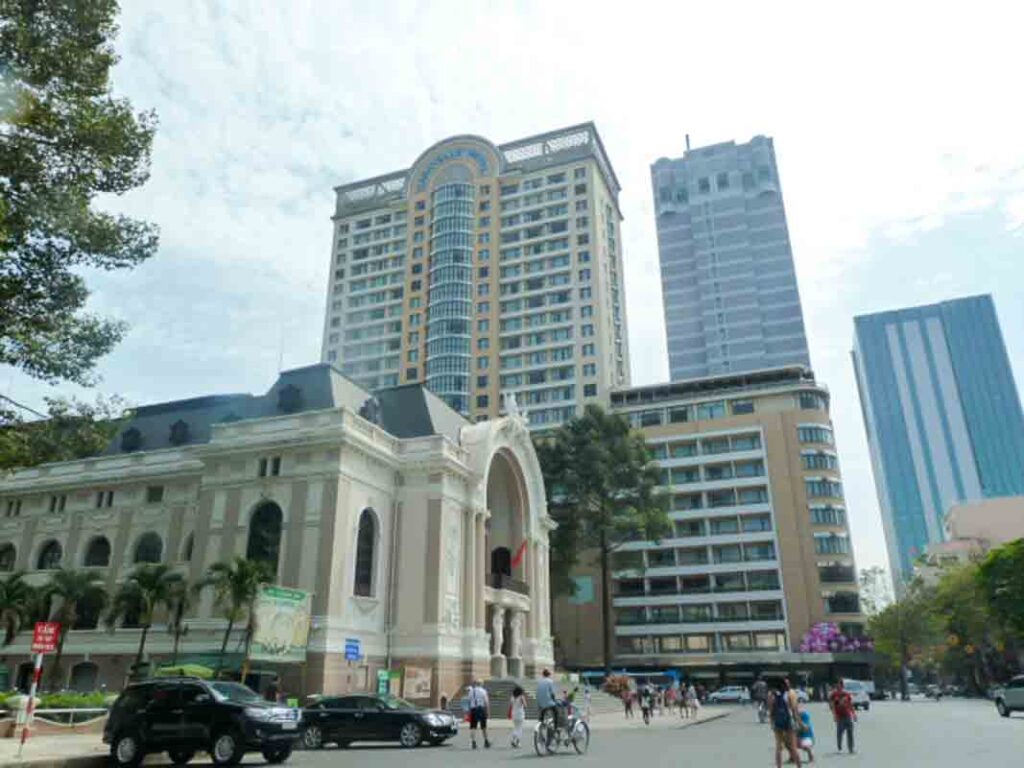This photograph captures a vibrant urban scene with both classical and modern architectural elements set against a bustling city backdrop. Dominating the left side of the image is a striking white, classical-style building, possibly a city hall or courthouse, featuring a large arched entryway and numerous arched windows. This building is flanked by a line of graceful palm trees along a sidewalk. In front, two black cars are parked, and people are seen walking and biking on the wide street that spans the center of the frame.

The scene transitions from the classical to the modern with a set of four buildings further back. The first of these is a tan, 10-story structure which appears residential, possibly an apartment complex. Towering behind and above it are three skyscrapers. The tallest one is distinguished by a rooftop balcony and a decorative half-moon element atop its roof. The second and third skyscrapers are simpler, tall rectangular buildings adorned with countless windows. 

On the right side of the photograph, there's a light brown building partially visible, with pink accents near its entrance, perhaps from signage or decorative elements. Trees intermingle with the buildings, adding a touch of nature to the urban landscape. The sky peeks behind the entire scene, providing a bright backdrop to this lively cityscape.